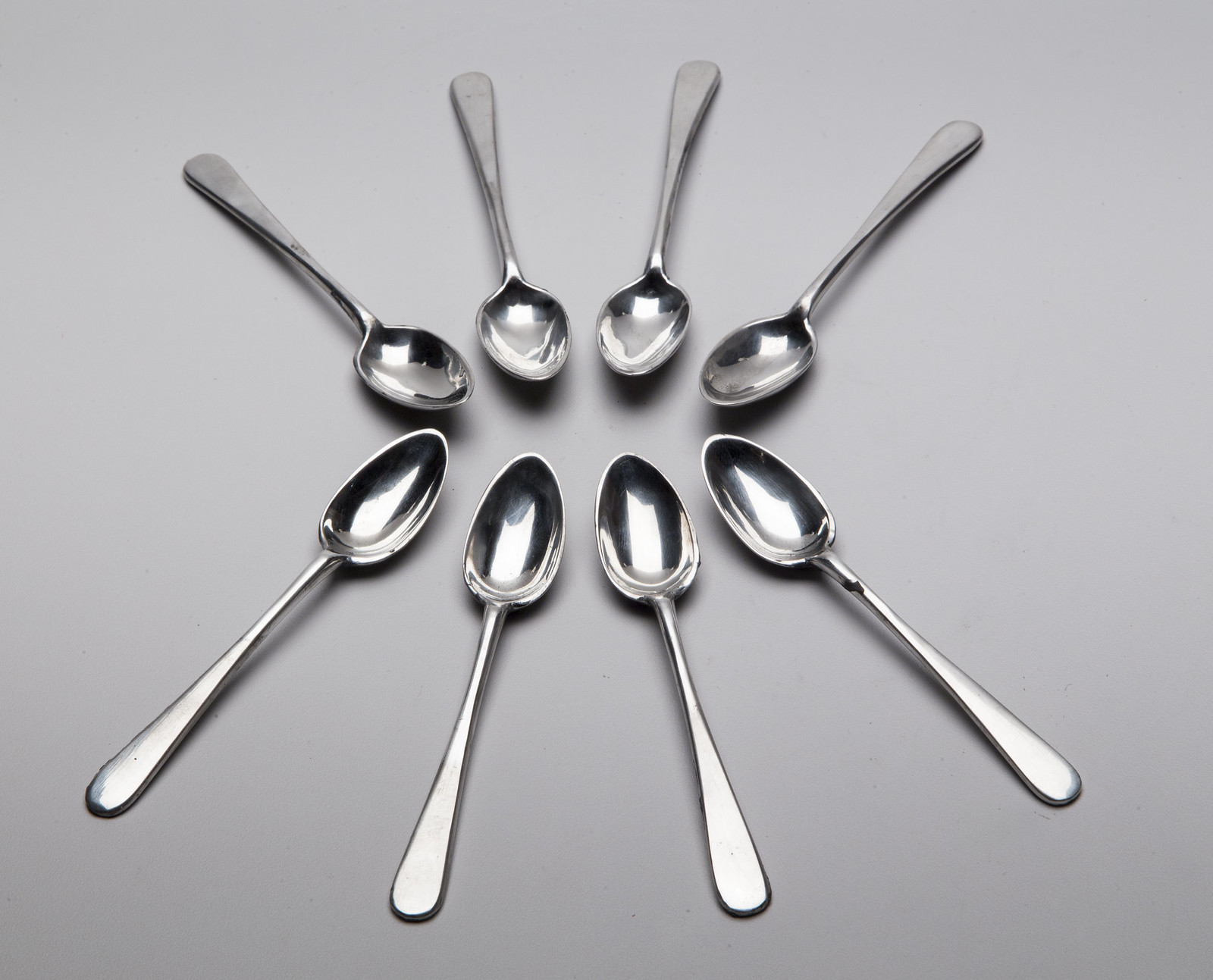The black and white image features a set of eight highly reflective metal teaspoons meticulously arranged on a medium gray background. They form an elliptical or oval shape with the bowls of the spoons facing inward towards a small empty space in the center. Each spoon is aligned symmetrically, creating an appearance similar to a sun or a floral pattern with their handles radiating outward. The top row comprises four spoons with the handles pointing upward, and the bottom row has handles pointing downward. The spoons appear to be identical with plain, flat handles, typical of a simple, unembellished design. A light source from above illuminates the scene, casting distinct square and oblong highlights in the bowls of the spoons, enhancing their silvery sheen. There is a slight darkening towards the bottom left corner of the background, possibly due to shading. Notably, a small black mark is visible on the stem of the fourth spoon in the bottom right, adding a subtle imperfection to the otherwise uniform set.